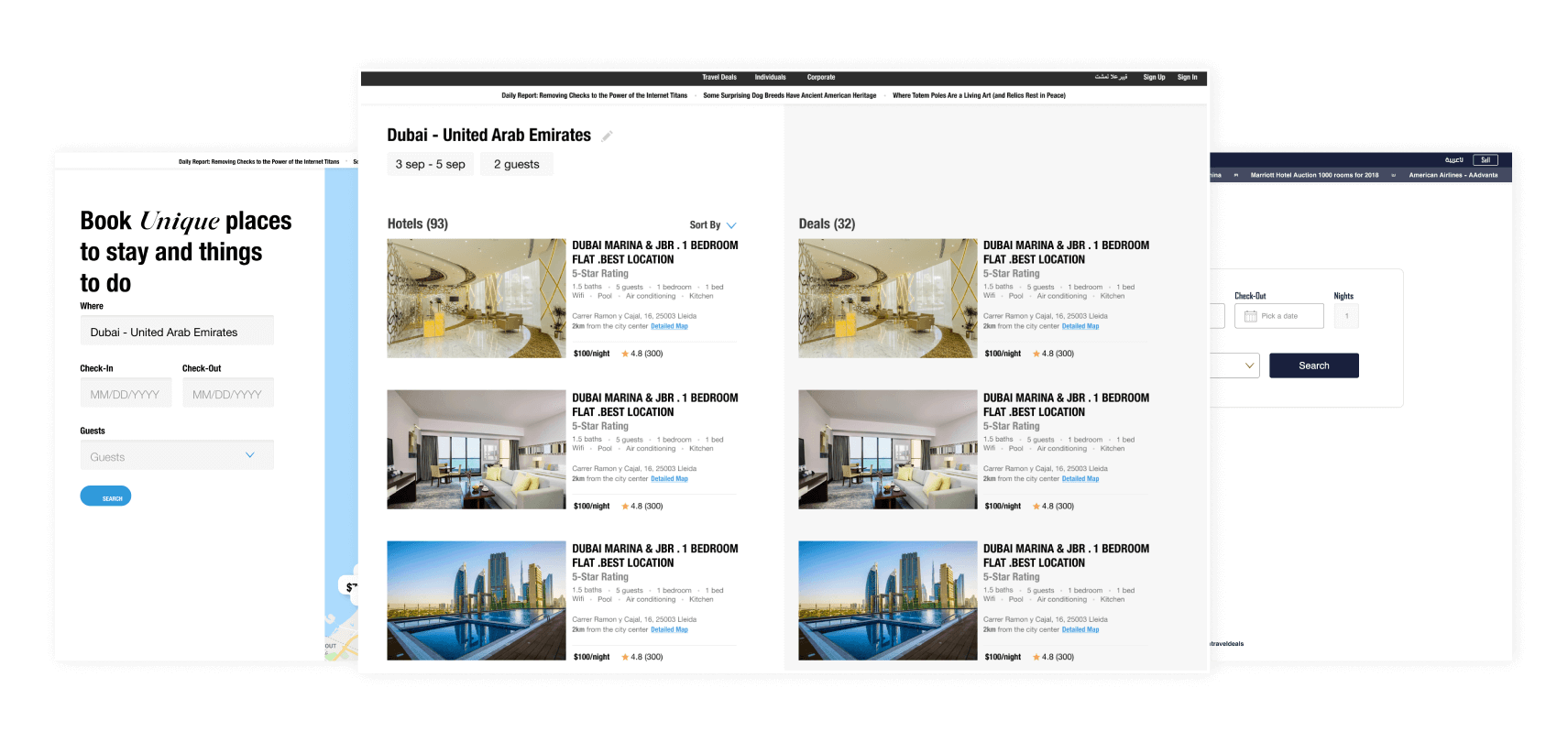The image is a composite of three panels from a website that promotes booking accommodations and activities, presumably targeting travelers. 

**Left Panel:**
The left panel features a promotional message encouraging users to "Book unique places to stay and things to do" in Dubai, United Arab Emirates. Below this message, the panel includes fields for selecting check-in and check-out dates, as well as the number of guests, although these fields are currently empty.

**Middle Panel:**
The middle section displays a black bar at the top, showing details of a search for accommodations in Dubai from September 3rd to September 5th, for two guests. The search yields 93 hotel options, with 32 of them offering deals. Below this bar, there are images and brief descriptions of specific accommodation options. One image showcases a view of the skyline, another features a living space, and a third displays a stairwell. Each listing is labeled "Dubai Marina and JBR one-bedroom flat best location."

**Right Panel:**
The right panel appears to be dedicated to searching for flights, although specific details about this search functionality are not provided.

Overall, the image suggests a user interface designed for booking both accommodations and flights, with a focus on trips to Dubai.